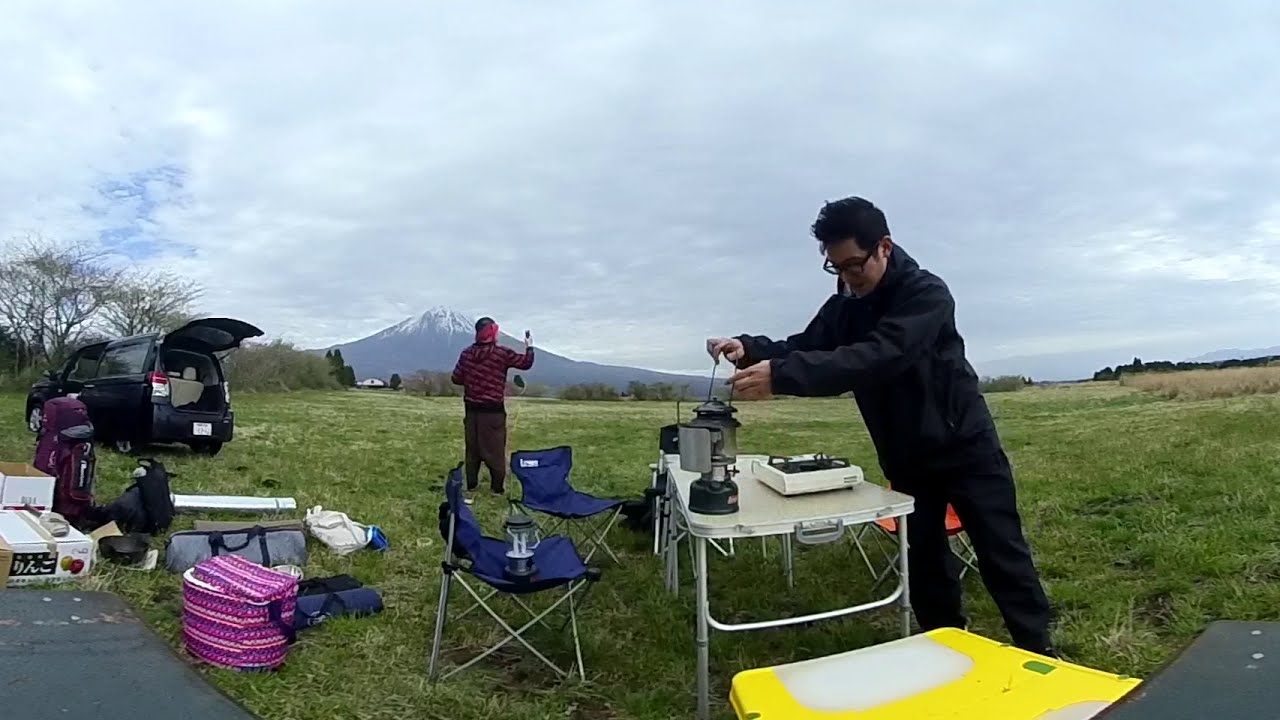In this detailed image, we see a vibrant outdoor camping scene set on a grassy field with a picturesque backdrop of what appears to be Mount Fuji, capped with snow. The scene is bustling with activity as two men are in the midst of setting up their camping equipment. 

The man closer to the foreground, dressed in a black outfit with a jacket, is attending to a lantern and a portable cooker on a table. Nearby, a couple of blue camping chairs are strategically placed, one of which has another lamp sitting on it. Scattered around the campsite are multiple bags, including a gray bag, a magenta bag resembling a golf bag, and other assorted gear and boxes.

Further in the background, another man, dressed in red with brown pants, is photographing the surrounding majestic landscape. To his left, there is a black or dark navy SUV with its back latch and side doors open, suggesting it’s being unloaded. Surrounding the campers, the expansive green field extends into the distance, dotted with trees, while an overcast sky with patches of blue peeks through the clouds, providing a serene yet dynamic ambiance to this daytime camping adventure.